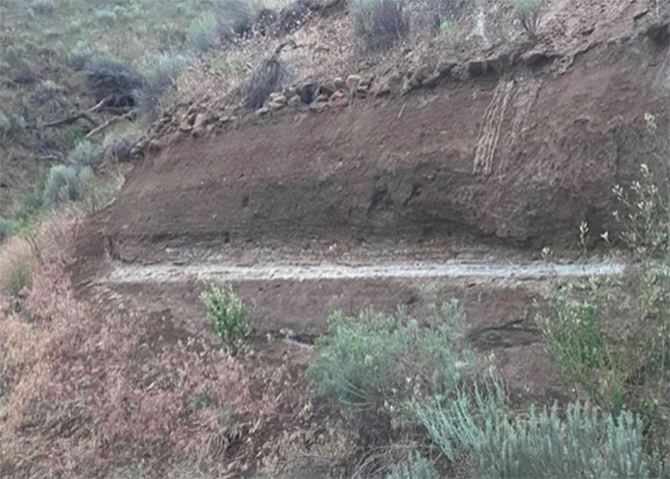The image depicts a bland, dry landscape featuring a flat, carved-out dirt surface, possibly the side of a hill or mountain. This area transitions into a slope adorned with sporadic, dull green plants, including bushes, weeds, and grass. At the base of the dirt wall, there's a questionable white line which might indicate a flat path or another carved-out section. The top of the flat surface is lined with a row of rocks, adding to the rugged terrain. Overall, the colors are unsaturated, contributing to the arid appearance of the scene, and the image is somewhat blurry, making specific details difficult to discern.